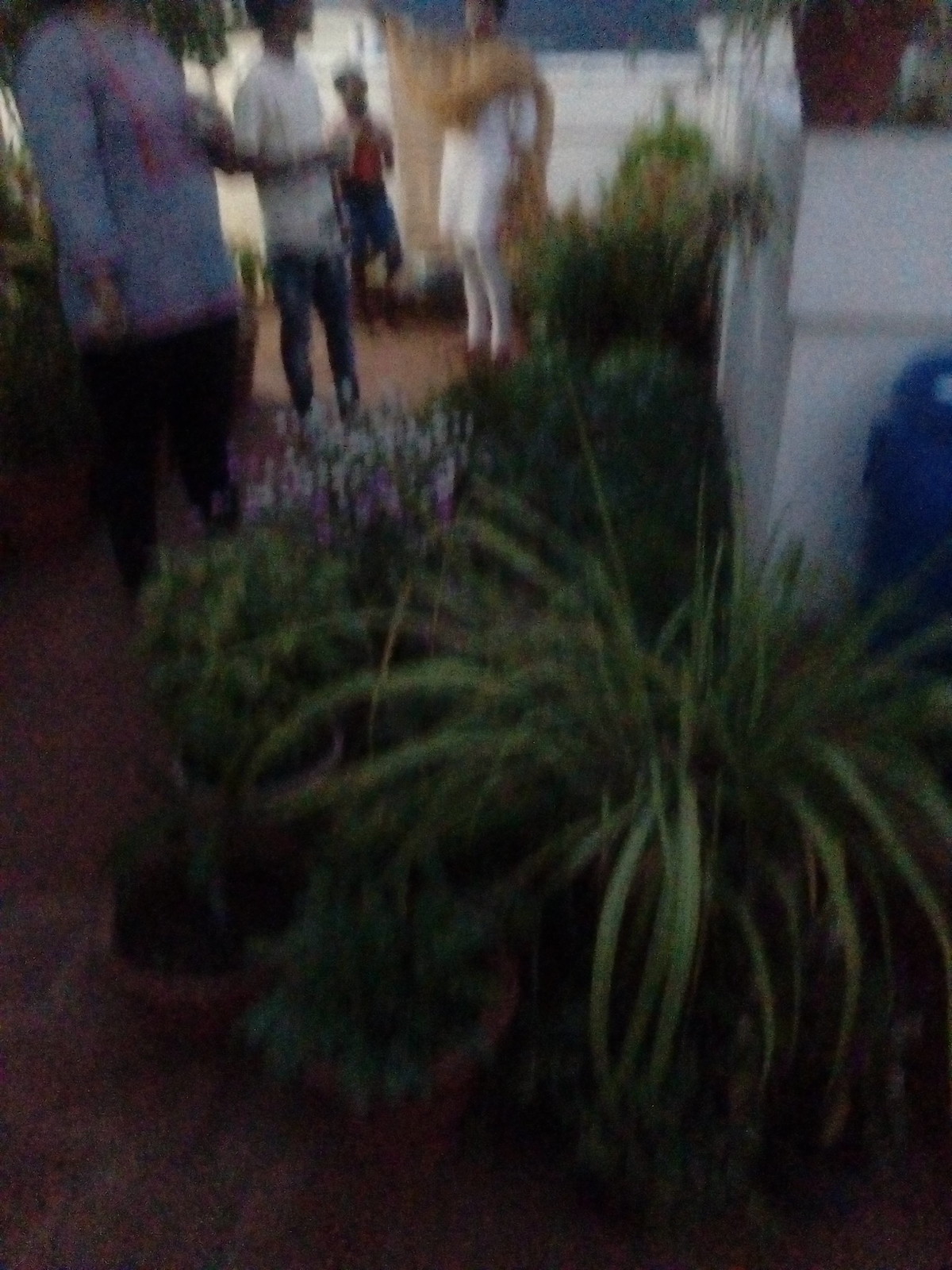In this blurry photograph taken in what seems to be a courtyard, the forefront is dominated by a lush collection of plants in containers. Central to the image are vibrant white and purple flowering plants, flanked by a green leafy plant. To the right, a plant resembling a fern or spider plant extends its stems outward, with its foliage cascading over the container sides. 

In the upper middle right section of the frame, a portion of a blue trash can is partially visible, positioned in front of a white wooden post. Moving further into the background towards the upper left, a group of people is gathered, engaged in conversation. One individual, dressed in a long-sleeved blue shirt with a distinctive red sash draped over their shoulders, is partially obscured, with their head not visible in the shot. This person is dressed in black pants. Next to them stands someone in a short-sleeved white collared shirt and jeans. Further back, another individual wears blue shorts, a red shirt, and a small white jacket. To the right of the group, a person who might be a bride is dressed in a white gown accompanied by white stockings.